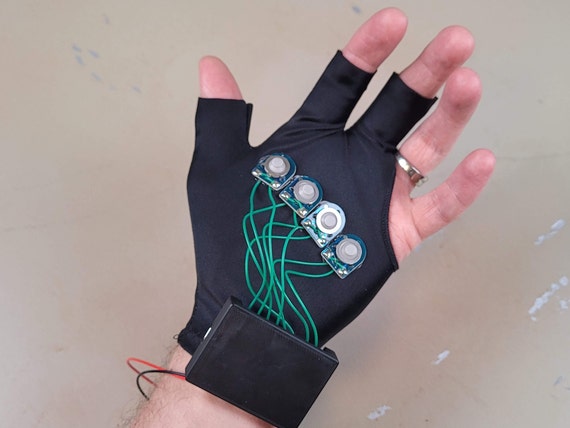The image features the left hand of a Caucasian man wearing a dark blue or black electronic glove with partial fingers, exposing the thumb, pointer finger, and middle finger, while the ring and small fingers are entirely covered. The glove includes intricate electronic components, most notably four clear plastic-encased discs with curved tops and flat bottoms, mounted on the palm. Each disc appears to be a sensor, equipped with a silver interior ring, and connected to a black rectangular box on the man's wrist via green wires. Two green wires link to each of the four sensors, and additional red and black wires extend from the box. The man has a silver wedding ring on his ring finger. The background is a white table with visible scratches and scuffs, adding a textured context to the scene. Subtle stripes and a beige tint are also present.